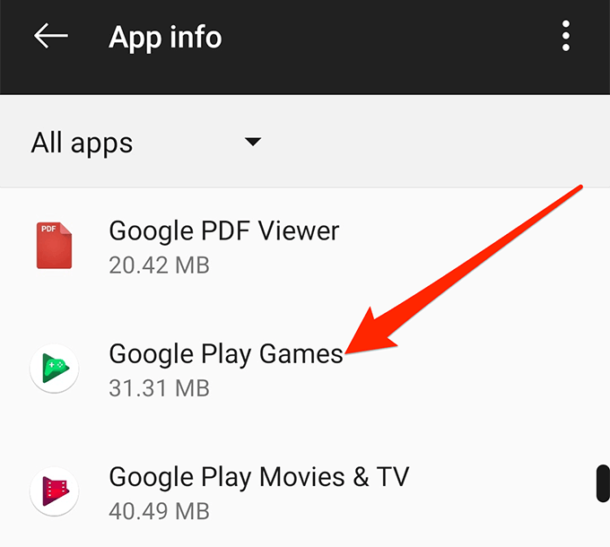This image is a screenshot taken on a mobile device. The screenshot itself has a roughly square shape, possibly slightly wider than it is tall. At the very top of the image is a black horizontal bar spanning from left to right. On the left side of this bar is a white left-facing arrow, and to its right is the white text "App info." Towards the right side of the bar, there are three white dots arranged vertically.

Immediately below this black bar is a light gray horizontal bar displaying the text "All apps" in black, accompanied by a black downward-pointing triangle. The background beneath this bar is a lighter shade of gray.

The main content consists of a list of three apps. The first app listed is "Google PDF Viewer," which has an icon resembling a red piece of paper with the letters "PDF" on it and a folded corner. This app takes up 20.42 megabytes of storage. The second app is "Google Play Games," with a logo featuring a white circle containing a green triangle and a green gaming console, using 31.31 megabytes of storage. The third app on the list is "Google Play Movies & TV," which has a logo that includes a dark reddish triangle and a red movie reel within a white circle, and uses 40.49 megabytes of storage.

A red arrow is pointing specifically at the "Google Play Games" app, emphasizing it among the listed apps.